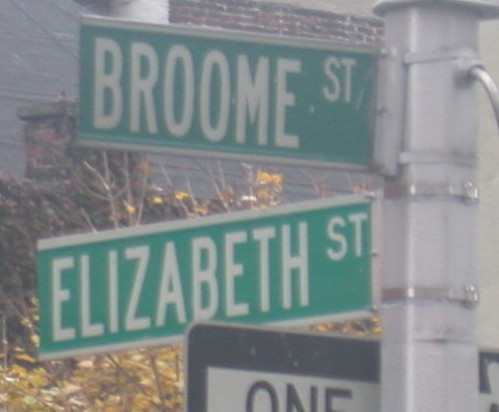This image depicts a set of traffic signs at an intersection. Prominently featured are two green street signs: one for "BROOM ST" and the other for "ELIZABETH ST," both in white, uppercase letters. The street names "BROOM" and "ELIZABETH" are notably larger compared to the smaller "ST" suffix on both signs. The signs are bordered by silver metallic frames and are mounted on a sturdy metal pole. Below these street signs, there is a black rectangular sign with a white arrow and the words "ONE WAY" indicating the direction of traffic flow.